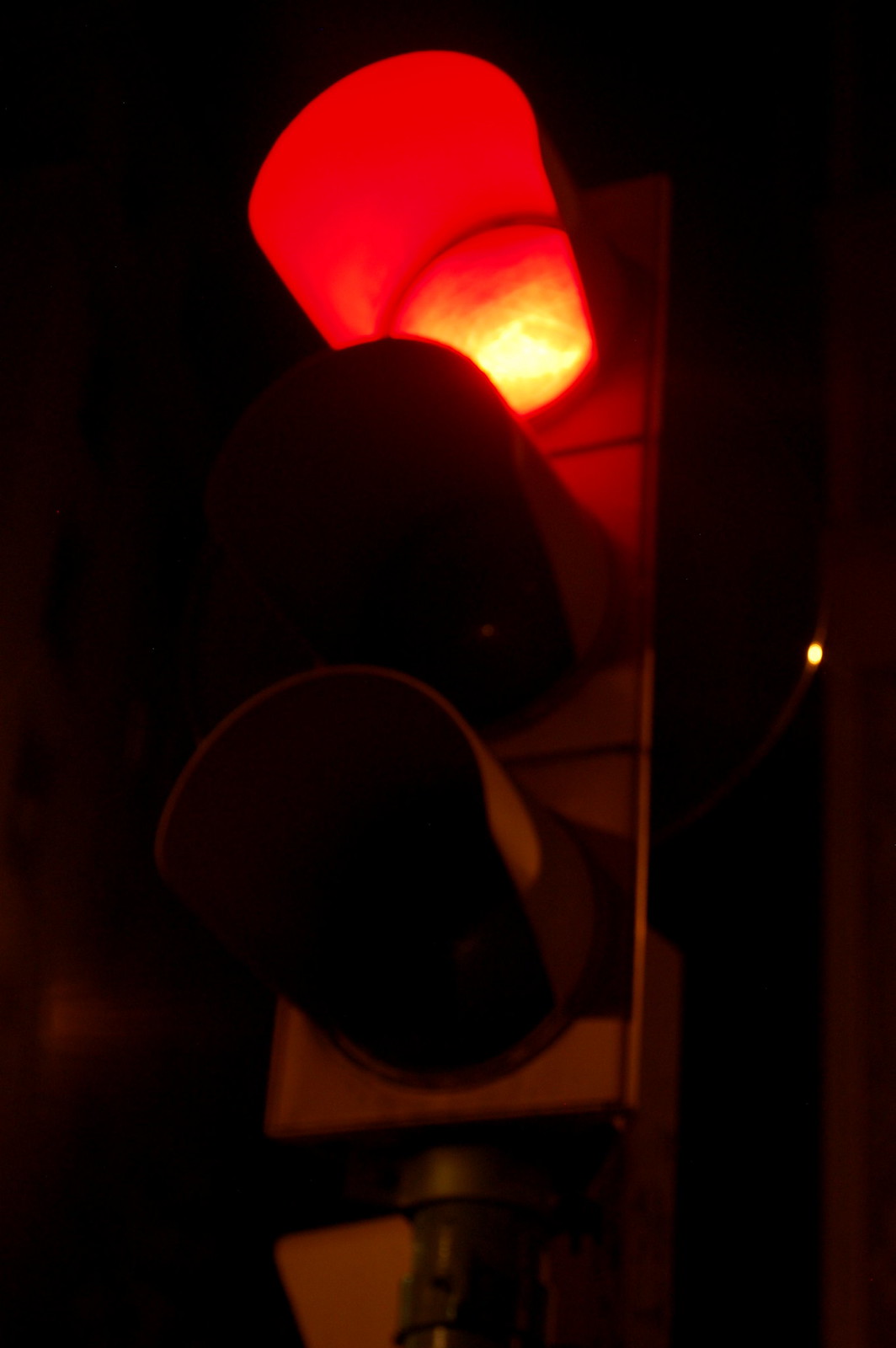A nighttime photograph captures a towering traffic light viewed from below, set against an almost pitch-black background. The red light glows intensely, casting a vivid hue that contrasts sharply with the darkness, while the adjacent yellow and green lights remain unlit. The prominent red hood encasing the lit bulb adds depth to the scene, forming a gradient from deep red to a radiant reddish-yellow at the center of the light. A small, mysterious yellow dot appears on the far right side of the image. Despite the enveloping darkness, the base of the traffic light structure is faintly visible, anchoring the composition.